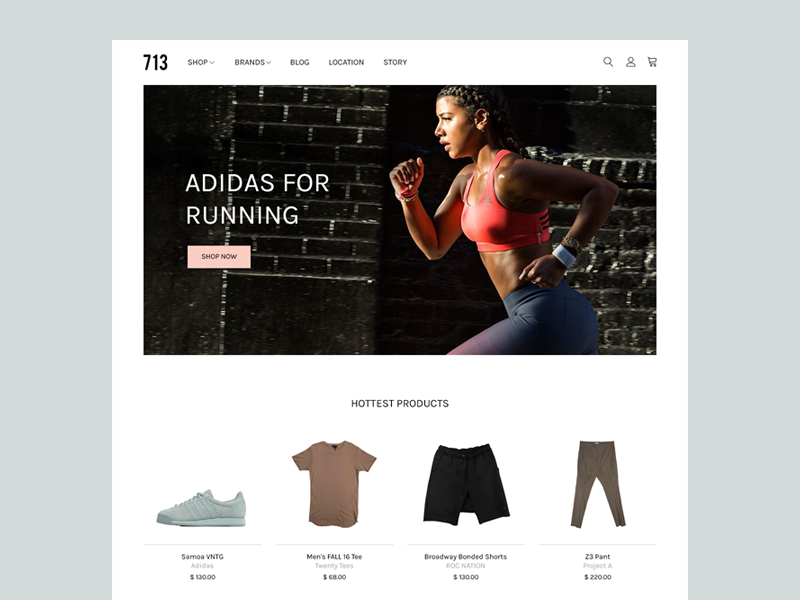Screenshot from the 713 Website:

The top left corner displays the website name, "713," accompanied by navigation buttons labeled "Shop," "Brands," "Blog," "Location," and "Story." Centrally positioned is a rectangular image featuring a fit Black woman mid-run. She is attired in a pink sports bra and blue sports pants, with her hair tied back in a braid, emphasizing her dynamic and athleticism. Adjacent to her, the text "Adidas for Running" is visible, along with a pink "Shop Now" button.

Below this image, there is a title that reads "Hottest Products." The first listed item is a "Samoa VNTG Adidas Shoe," priced at $130. Following this, the "Men's Fall 16 Inch Tee" is available for $65. The third item is "Broadway Bonded Shorts," priced at $130. Lastly, there are "Z3 Pants" which are offered for $220.